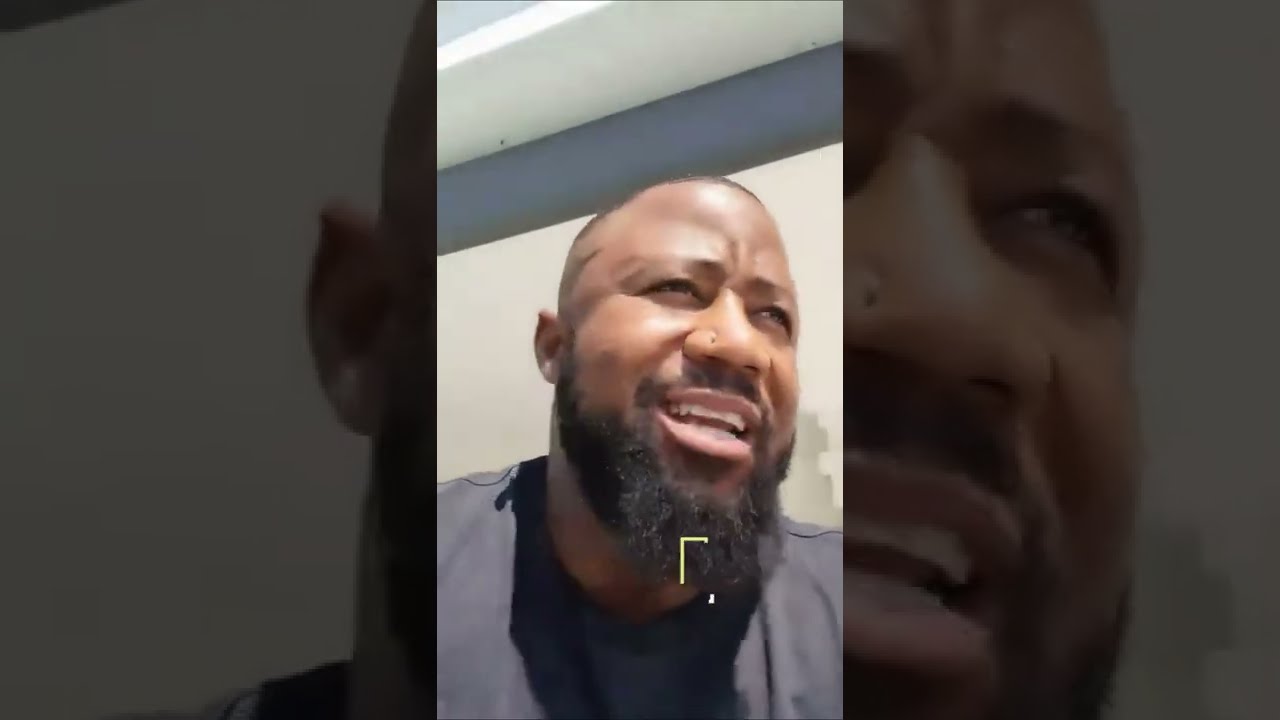This image features a wide rectangular layout with a centrally positioned tall rectangular portrait of an African American man. Flanking this central image are wider rectangular, close-up photos of different sections of the main portrait, all shaded darker for emphasis. The man, who appears to be part of a TikTok video or similar, is visible from the shoulders up, though his actual shoulders are cut off. His head is tilted slightly to the right, and he is making a somewhat confused yet happy expression with his mouth open, revealing both rows of teeth.

He has short, shaved dark brown hair and a thick, black beard with a matching mustache. Notably, there is a small hole in his nose where a piercing might have been. The background shows he is outside, possibly near a white building with a gray top or a blue stripe at the top and a white awning. He is wearing a navy blue, bluish-gray, or black shirt, with the shadow of his beard casting down the middle of it. Additionally, a bright yellow line, shaped like an upside-down 'L', is positioned prominently in front of his beard, adding a striking element to the image. The setting is clearly daytime, emphasizing the details on his face and attire.